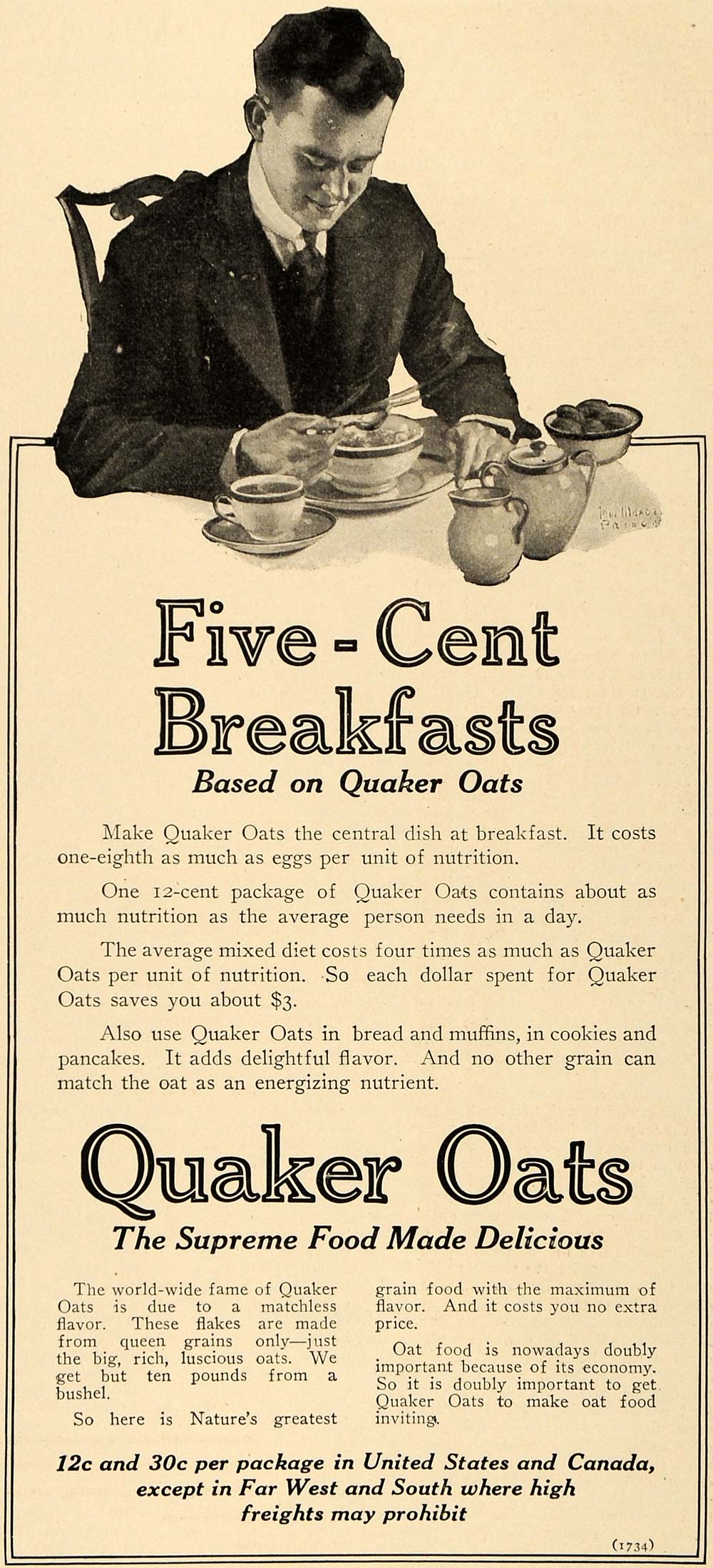This vintage sepia-toned Quaker Oats advertisement appears to be from the 1930s or 1940s and promotes a five-cent breakfast. At the top of the ad is an image of a well-groomed man dressed in a black suit, white collared shirt, and black tie, sitting at a wooden dining table. He has short, neatly trimmed hair and is enjoying a bowl of oatmeal while holding a cup of coffee. The table is set with additional items, including a bowl that possibly contains strawberries, a plate, a teapot, and other utensils.

The main headline reads, "Five Cent Breakfast," and suggests making Quaker Oats the central dish at breakfast for its cost efficiency and nutritional value. The ad boasts that one 12-cent package of Quaker Oats contains about as much nutrition as an average person needs in a day and costs one-eighth as much as eggs per unit of nutrition. Additional paragraphs extol the economic benefits of Quaker Oats, highlighting that opting for this breakfast staple can save consumers significant amounts of money.

The advertisement also mentions that Quaker Oats can be used in a variety of foods, including bread, muffins, cookies, and pancakes, all while maintaining a delightful flavor unmatched by other grains. The bottom section of the ad details the pricing: 12 cents and 30 cents per package in the United States and Canada, except in the far West and South where high freight costs may apply.

The ad concludes with the tagline, "Quaker Oats: The Supreme Food Made Delicious," underscoring the product's matchless flavor and economic benefits.